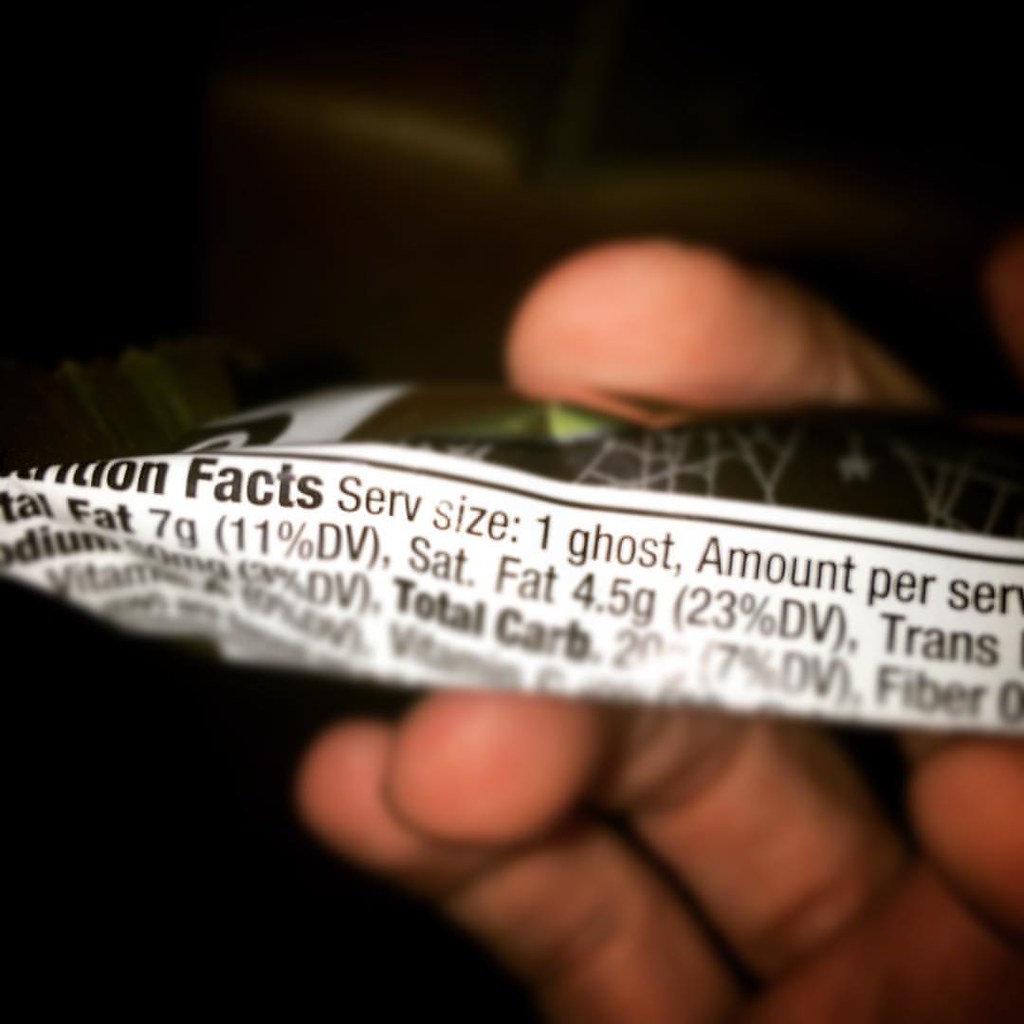The image is a close-up, color photo of the nutrition facts on the side of a Halloween-themed food package, with a blurred, dark background. The photo prominently features a person's right hand, palm down, with their pinky, ring finger, and middle finger visible. The middle finger is positioned on the top of the bag, while the other fingers rest on the bottom. The index finger is slightly lifted, showing part of the palm but not the full hand.

The nutrition label details that the serving size is listed as "one ghost," likely indicating this is a piece of Halloween candy shaped like a ghost. The package also features a spiderweb design with possible bat motifs, suggesting a spooky, festive theme. Key nutritional information visible includes:

- Total Fat: 7 grams (11% DV)
- Saturated Fat: 4.5 grams (23% DV)
- Trans Fat: (partially cropped)
- Total Carbohydrates: 29 grams (7% DV, partially cropped)

Some of the vitamin information is illegible, but the overall context strongly suggests that this is a nutritional label for a Halloween candy product.